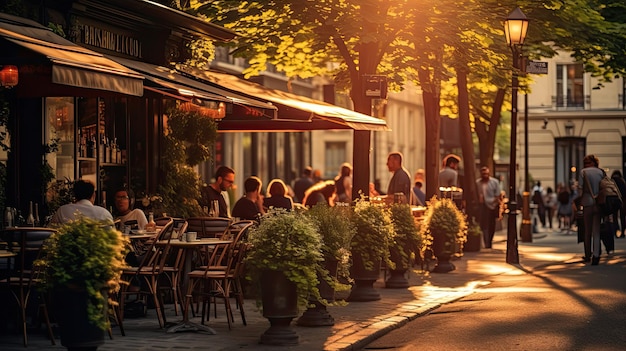This vibrant and clear photo captures a bustling city street bathed in sunlight, casting dynamic shadows on the ground. The scene is characterized by a lively bistro with a black awning, where patrons enjoy meals at outdoor tables adorned with overflowing black planters. The street is animated with people walking on the sidewalks and in the street, creating a busy, summery atmosphere. The thoroughfare is lined with mature trees sporting green foliage and flanked by classic yellowish buildings, as well as a historic-looking white building in the background. Older-style lamp posts add to the charming, picturesque ambiance, reminiscent of an old, historic city like Philadelphia. The sunlight filters through the trees, enhancing the idyllic setting as people relish the pleasant weather.